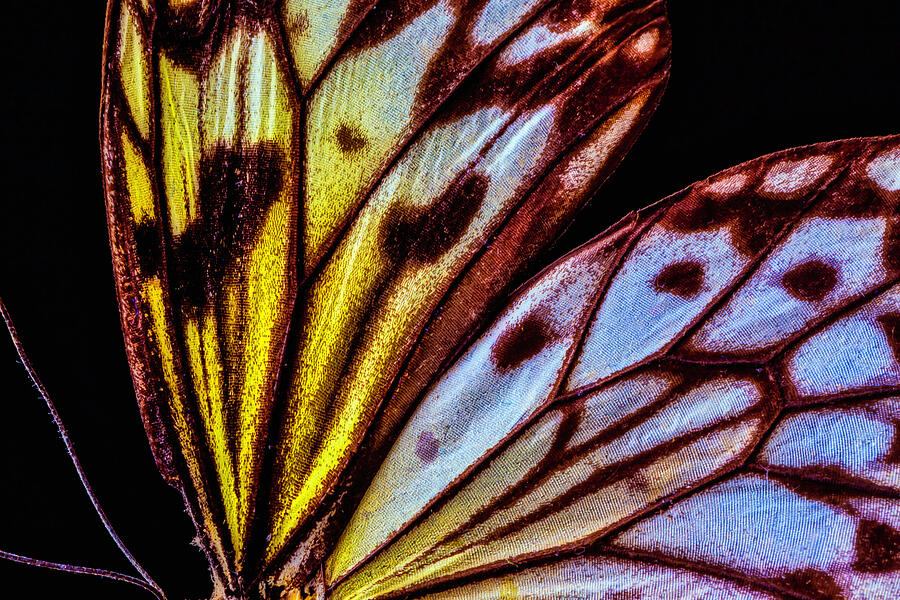The image depicts an extremely close-up, full-color view of what appears to be butterfly wings against a stark black background. The rectangular image highlights the delicate, intricate details within the wings, showcasing an array of colors transitioning from pale blue to vibrant yellow, adorned with distinctive black spots and decorative veins or stems. The horizontal edge of the image is the longest, emphasizing the expansive, delicate nature of the wings. In the lower corners, though partially cut off, you can discern the faint outline of what seems to be the butterfly's antennae, further signifying its insect origin. The close-up perspective reveals the wings' fragile beauty and the complexity of their design, making the subject's graceful allure the focal point of the image.